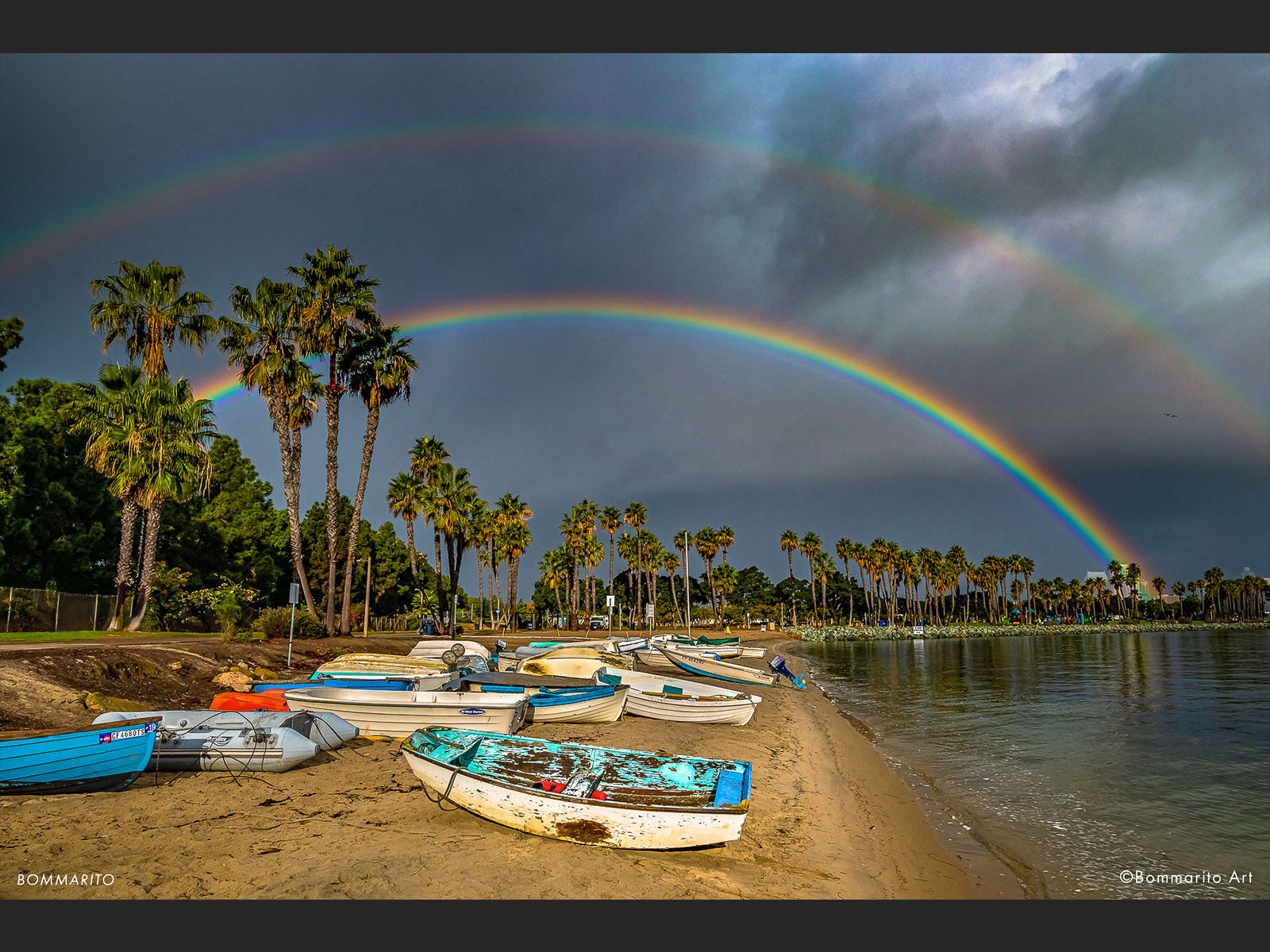This stunning outdoor daylight photograph captures a remarkable double rainbow arcing over a tranquil beach. The beach, featuring dark brown sand, stretches vertically through the center of the image. The sky above is densely overcast with black and gray clouds, hinting at a recent storm. The lower rainbow is vivid and bright, showcasing distinct bands of blue, yellow, orange, and red hues, while a fainter, second rainbow arcs gracefully above it. The water on the right side of the photograph is still and has a dark greenish tint, with minimal wave action. Along the shore, multiple small boats of various colors—including white, blue, and yellow—are drawn up and lined on the beach. These boats appear to be small rowboats with motors, easily maneuverable by a single person. On the left side, a line of lush palm trees curves gently toward the back right, following the shore's arc. The silky foliage of the trees frames the serene scene beautifully. In the bottom corners of the image, the name "BOMMARITO" and "copyright BOMMARITO ART" indicate the photographer responsible for capturing this breathtaking moment.